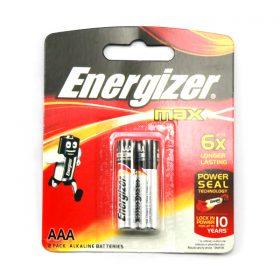The image features a blister pack of Energizer AAA alkaline batteries. The packaging is predominantly black with accents of red and yellow. There are two AAA batteries in the pack, each prominently displaying the Energizer brand name. The pack includes a hanging hole at the top for easy display on retail hooks or nails. The batteries themselves are colored in black, red, and white. The packaging highlights key features such as "Energizer Ultimate Lithium," indicating that these batteries last up to six times longer than ordinary batteries and can retain power for up to 10 years.